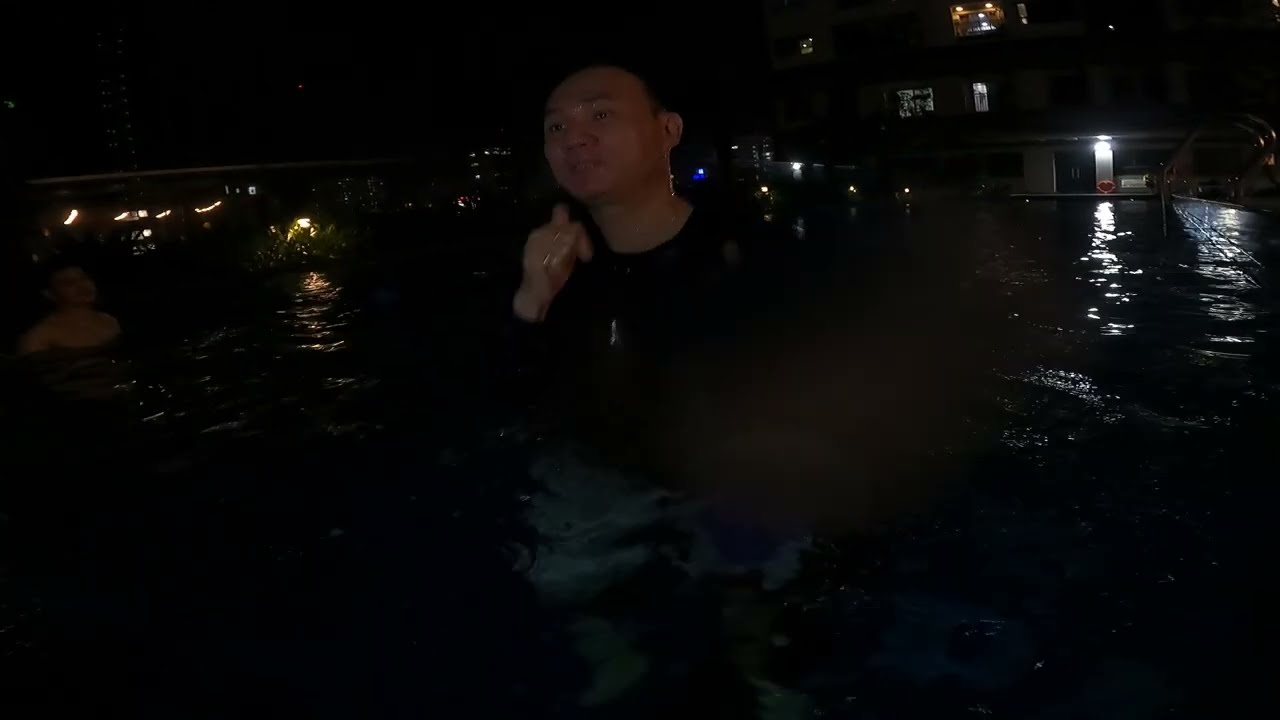In this somewhat blurry nighttime photograph, the scene is dominated by an outdoor swimming pool under a pitch black sky. A multi-story building with sparse lighting looms in the background, possibly an apartment complex or hotel, while distant rectangular buildings with minimal illumination create a subtly urban atmosphere. Central to the image is an Asian man with short black hair, wearing a black t-shirt and blue swim trunks, standing in the pool. He has his right hand near his face, looking off to the left. Another man, shirtless and visible to just below his shoulders, is positioned on the far left, seemingly looking towards the central figure. Silver handrails line the pool's edges, glinting subtly in the sparse ambient light, adding a touch of detail to the composition.